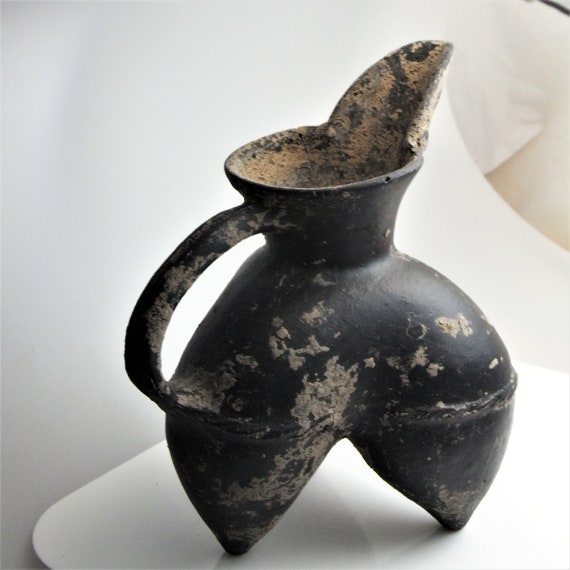Displayed on a white table, possibly in a museum setting, this ancient, weathered pottery piece stands as a testament to historical craftsmanship. The pottery is a dark, earthen brown color with noticeable pitting in light tan and yellow hues, indicating its age and the material's exposure over time. Notably, a large handle arches from the top rim down to about the middle of the artifact, complemented by a long, pointy spout for pouring liquids. The bottom is uniquely designed with two sharp, triangular legs forming a V-shape, which supports the vessel on the table. The artifact also shows signs of wear with white markings and what appears to be rust or paint chipping off. Furthermore, lines at the bottom reveal how the pieces have been melded together, showcasing the intricate details and historical significance of this pottery pitcher.